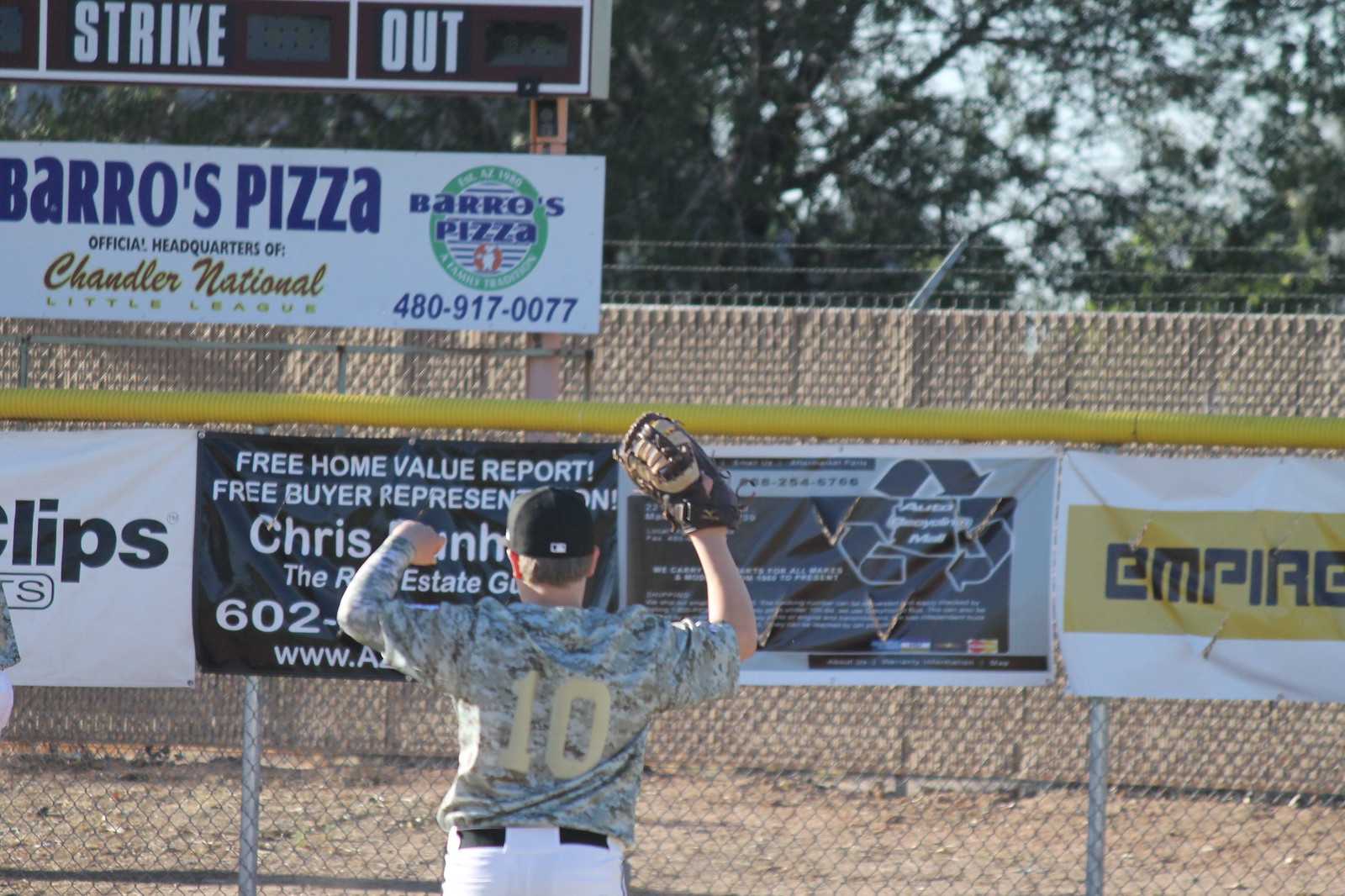A young baseball player, wearing a camouflage-patterned jersey with the number 10 in gold, stands with his back turned. He's clad in white pants and holding a brown glove high above his head with both hands, as he looks intently towards the outfield. The scene captures a sunny day on the baseball field, adding a warm and vibrant feel to the moment. The backdrop features a tan wall adorned with various small business advertisements, including "Barrios Pizza," "Great Clips," and other partially visible signs. Behind him, a white sign with blue lettering and a black scoreboard with "Strike It Out" in white writing are clearly visible. The player stands upright on the grass, seemingly poised and focused, while the day’s game, whether it's in progress or not, remains ambiguous.